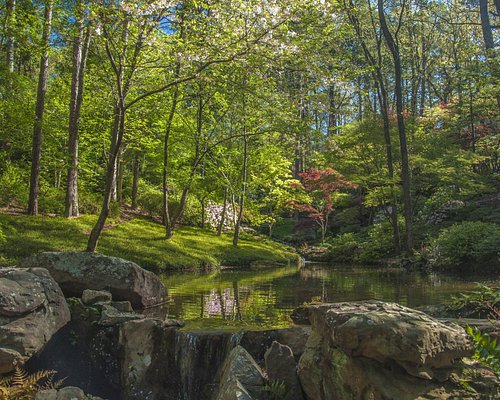This outdoor photograph captures a serene forest scene during springtime, characterized by a calm stream flowing through the center, which reflects the surrounding foliage. In the foreground, several large, tan and gray rocks are stacked up, creating a small waterfall that spills into the stream. The water appears to be a murky green, reflecting the lush greenery and trees above. To the left, there's a grassy area along the water's edge with young, short grass, and nearby bushes with blooming white flowers.

In the background, various trees populate the scene, including some with tall, skinny trunks adorned with fresh spring leaves. A tree with red leaves stands out on the right side, alongside others with pink and yellowish foliage. The sky peeks through the canopy, offering a glimpse of blue amid the verdant landscape. The right side of the image features a small hill rising among the trees and more patches of white flowers breaking the green monotony.

Overall, the picture exudes calmness and tranquility, presenting a rich mixture of natural elements like rocks, water, and diverse flora. This picturesque woodland is vibrant with life, depicted under a bright daytime sky, and embodies the serenity of a peaceful river flowing through a dense, blossoming forest.